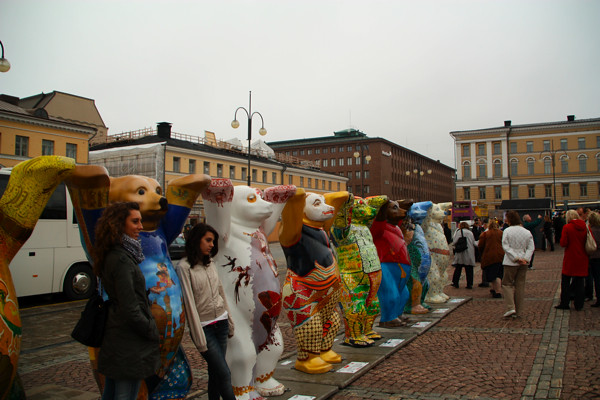The photograph captures an intriguing outdoor art display set in a European city square on a cloudy, cool day. The focal point is a line of approximately ten colorful, extravagantly decorated bear sculptures, each standing on its hind legs with paws raised and touching, resembling a procession of joyful teddy bears. These bears are individually adorned in vivid colors and unique designs — one is white with intricate patterns, another blends green and yellow hues, while yet another features blue and red tones. Their bodies showcase a variety of decorations, some with almost tribal, African-like motifs. Each bear sculpture is accompanied by a white placard at its feet, likely detailing the artist and the design.

In the background, a picturesque urban scene unfolds. The setting is a cobblestone street lined with quaint three-story buildings, painted in shades of orange, light orange, brown, and lighter brown. The sidewalk is a charming patchwork of small red bricks framed by gray bricks arranged in a square pattern. Old-fashioned lampposts with dual bulbs add to the historic ambiance. Amidst the sculptures, regular city-goers clad in long sleeves and sweater jackets, suggestive of the cool weather, stroll by or pose with the bears, including a little girl in a tracksuit with black hair, who stands out for her interaction with one of the statues. The scene is lively with an array of casual pedestrians, enhancing the feeling that this is a bustling, tourism-friendly area rich with cultural displays.